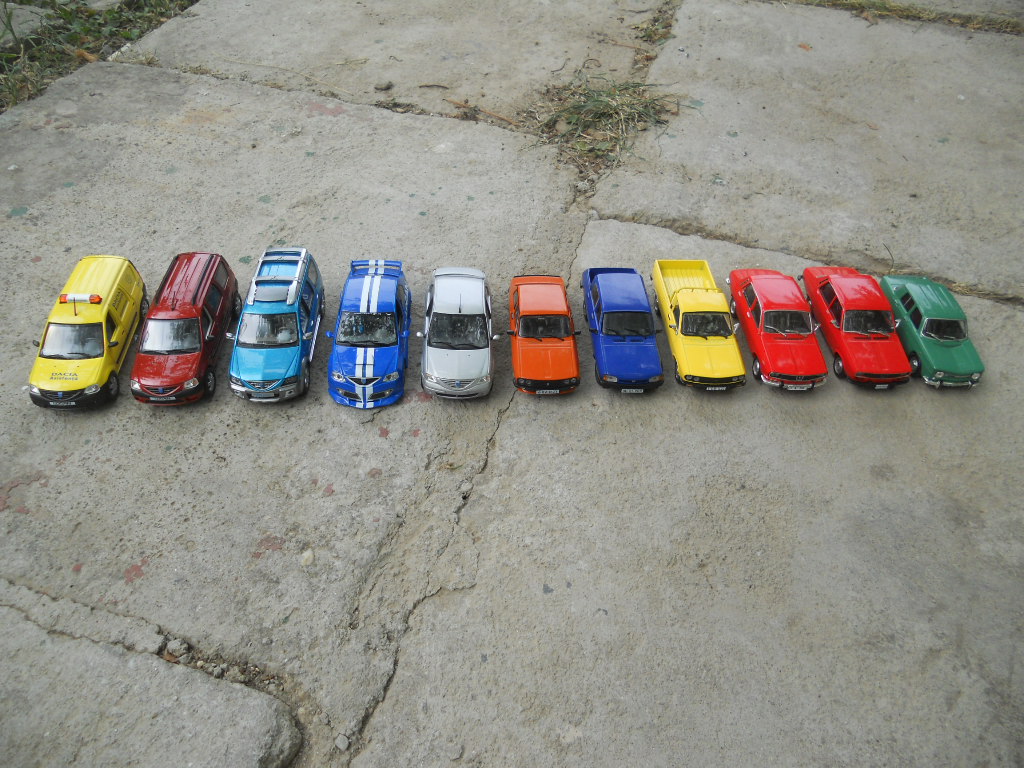The image is a color photograph taken outdoors during the day, offering a top-down view of a coarse stone or patio surface with dirt and grass sprouting between the cracks. The surface appears rustic and unpolished, likely made of concrete slabs. Under bright sunlight, a row of 11 colorful toy cars, possibly Hot Wheels or Matchbox cars, is lined up from left to right in the center of the image, all facing the viewer directly. Starting from the left, the cars include:

1. A yellow ambulance or van with lights mounted on the roof.
2. A maroon or red van.
3. A bright turquoise minivan with a roof rack.
4. A blue race car with double white stripes running from the spoiler, over the roof, and down the hood.
5. A silver or grayish sedan.
6. An older model brown muscle car.
7. A blue pickup truck similar to the orange one.
8. A yellow long-bed pickup truck.
9. Two red sporty sedans.
10. A green sedan, possibly reminiscent of an old Lada.

The colorful array of toy cars creates a vibrant contrast against the textured stone and grass background.